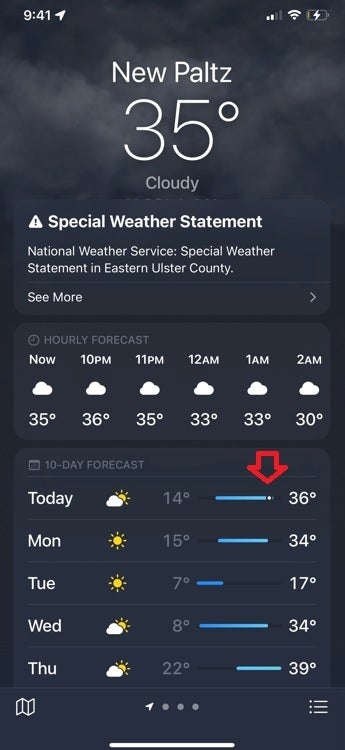In the provided screenshot of a weather application, taken at 9:41, several details are visible indicating device status and weather conditions for New Paltz, New York. The phone has two bars of carrier service, enabled Wi-Fi, and a low battery currently charging, as evidenced by the yellow battery indicator.

The weather status is prominently displayed, showing a temperature of 35°F with cloudy conditions. A special weather statement from the National Weather Service is highlighted, alerting about conditions in Eastern Ulster County. The application's visual design includes cloudy weather graphics against a dark backdrop.

The hourly forecast predicts slight fluctuations in temperature: 35°F at 10 p.m., 36°F at 11 p.m., 35°F at midnight, 33°F at 1 a.m., and 30°F at 2 a.m. Additionally, the 10-day forecast is detailed, with an arrow indicating a downward trend in temperature. Today's high is 36°F. Future days are forecasted to be sunny but cold: Monday with a high of 34°F and a low of 15°F, Tuesday with a high of 17°F and a low of 7°F, and Wednesday showcasing a warmer high of 34°F.